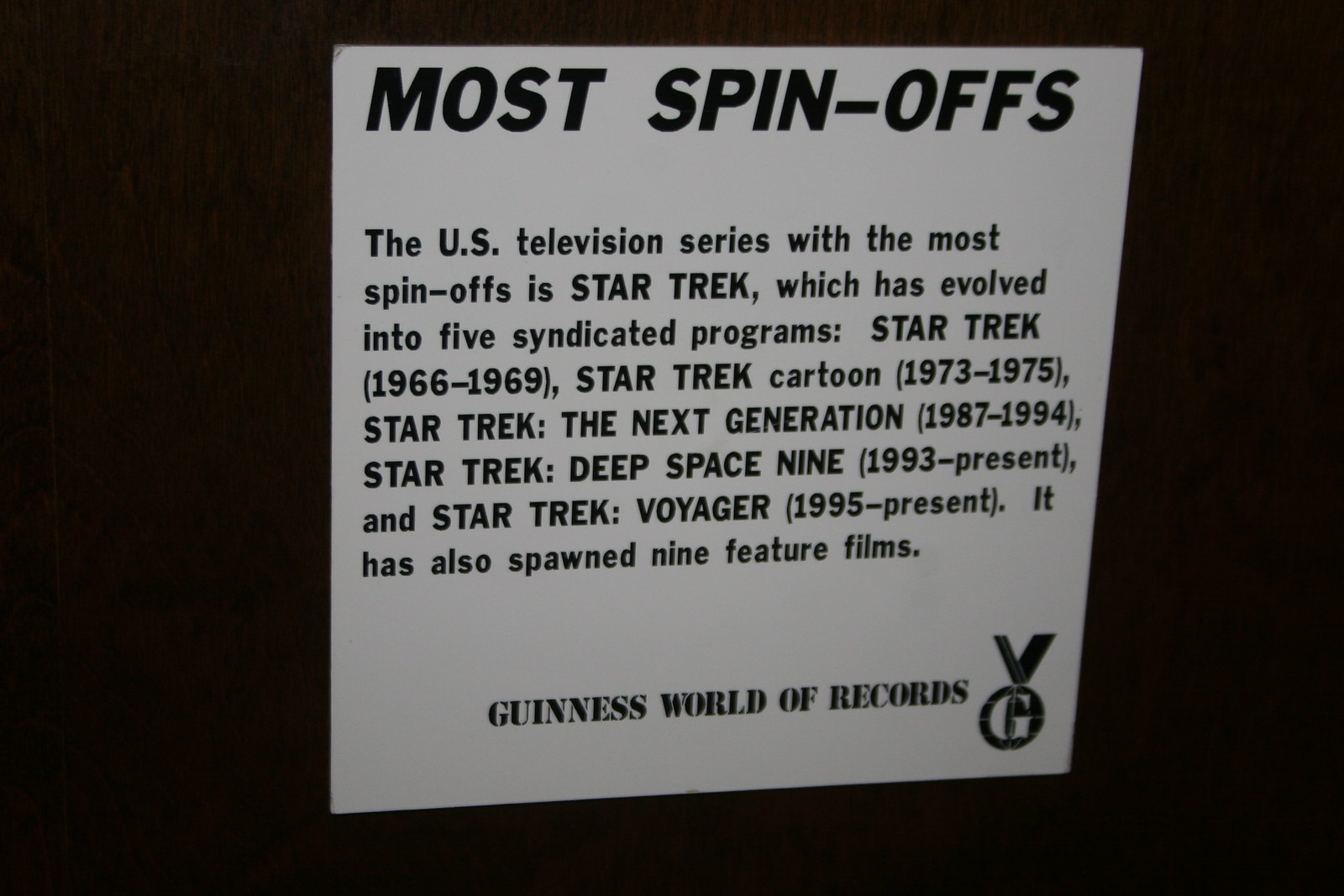The image depicts a plaque from the Guinness World Records, set against a mostly black background. At the top, bold black text reads "Most Spinoffs," emphasizing the record being awarded. Below, a detailed paragraph states that the U.S. television series with the most spinoffs is Star Trek. Specifically, it has evolved into five syndicated programs: Star Trek (1966-1969), Star Trek: The Animated Series (1973-1975), Star Trek: The Next Generation (1987-1994), Star Trek: Deep Space Nine (1993-present), and Star Trek: Voyager (1995-present). Additionally, the series has spawned nine feature films. A Guinness World Records logo, resembling a medal with a large "G," is present at the bottom of the plaque. This record appears to have been recognized in the late 1990s, as indicated by the dates mentioned. The overall design of the image is stark with the white plaque's detailed text taking up most of the visual space on the black background.